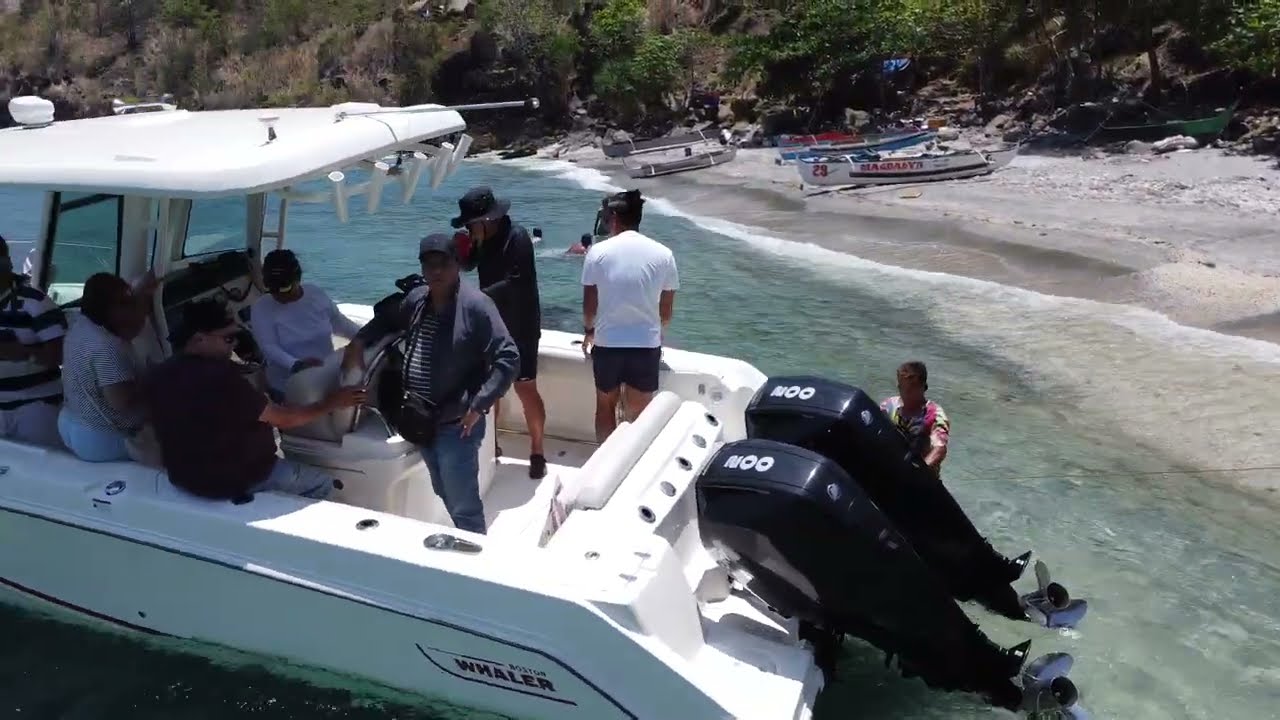The image depicts a lively scene at a boat launch area. Dominating the left foreground is a large white powerboat with the name "Whaler" visible on its side and twin 200 horsepower black engines at the stern. Inside the boat, eight people are engaged in conversation, with most wearing white or black shirts, black hats, and one in light blue jeans. Close to the boat, a man stands in the shallow, bluish-green water, appearing to work on the engines. The shoreline features tan and brown sand, with four small canoes scattered along it, displaying a mix of colors including red, blue, black, and white. The upper half of the image is filled with green trees against a hilly backdrop, under a sunny sky.